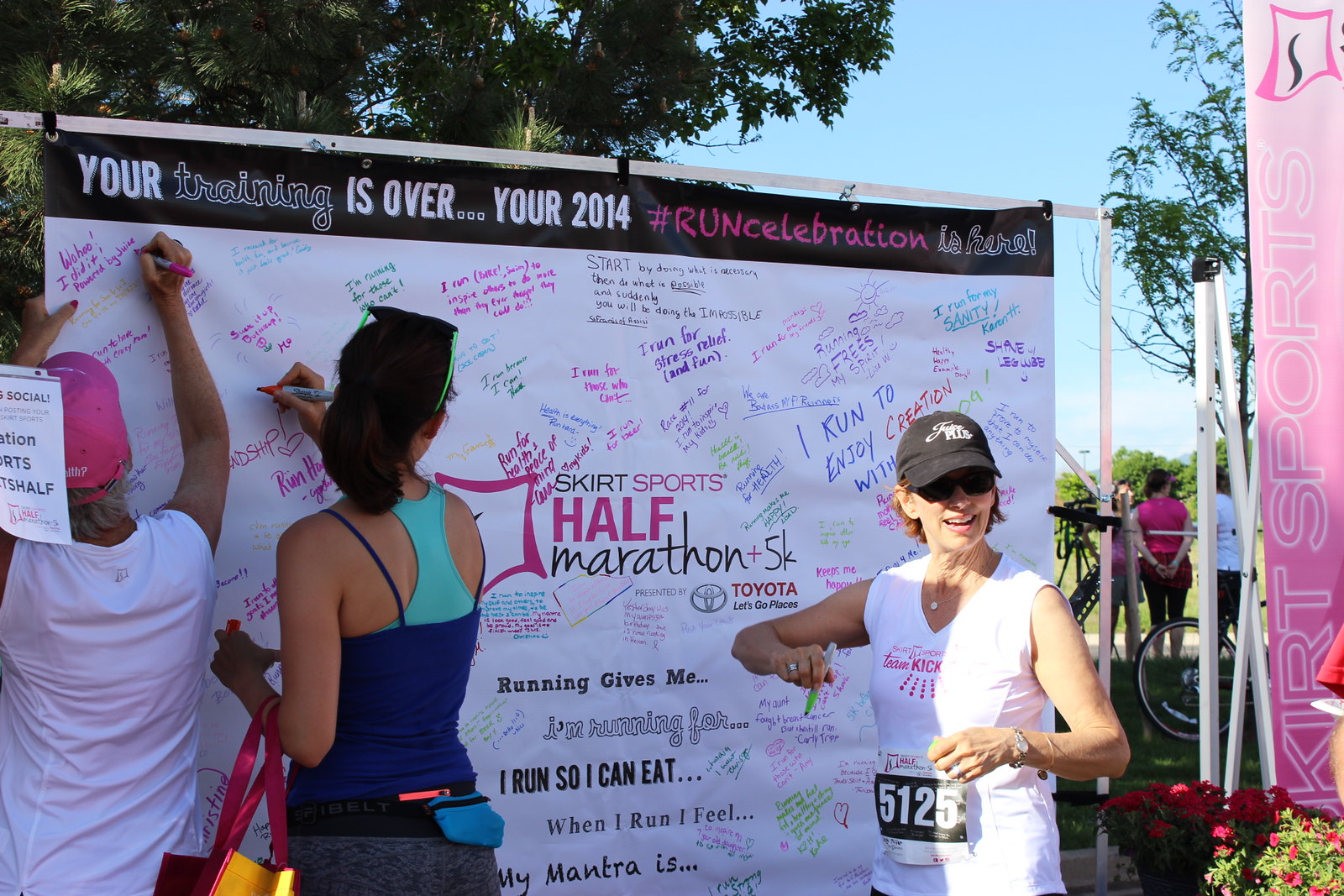In an outdoor setting with a clear blue sky visible through the leaves of nearby trees, three women stand in front of a large banner attached to a white frame. The banner reads, "Your training is over. Your 2014 Hashtag Run Celebration is here," and is covered with numerous signatures and messages. Central on the banner is the text "Skirt Sports Half Marathon Plus 5K" alongside the Toyota logo and slogan, "Let's Go Places."

The woman on the left, with her back to the camera, wears a white tank top and a pink hat and is using a pink marker to sign the banner. To her right, another woman, also with her back to the camera, is preparing to autograph the banner. She is dressed in a blue tank top with an aqua sports bra underneath, gray shorts, and has her hair tied up. She is holding a red marker and wears green-framed sunglasses. The woman on the far right faces the camera, slightly angled to her left. She is wearing a white tank top with the number 5125 on it, a black hat, and is holding a green Sharpie marker. Her left hand, which sports a watch, rests in front of her body. 

In the background, beyond the banner, several other people can be seen, including one in a pink shirt and another in a light shirt. The right side of the image also shows some rose bushes. The scene clearly captures the celebratory and communal spirit of the event, taking place under a bright and cloudless sky.